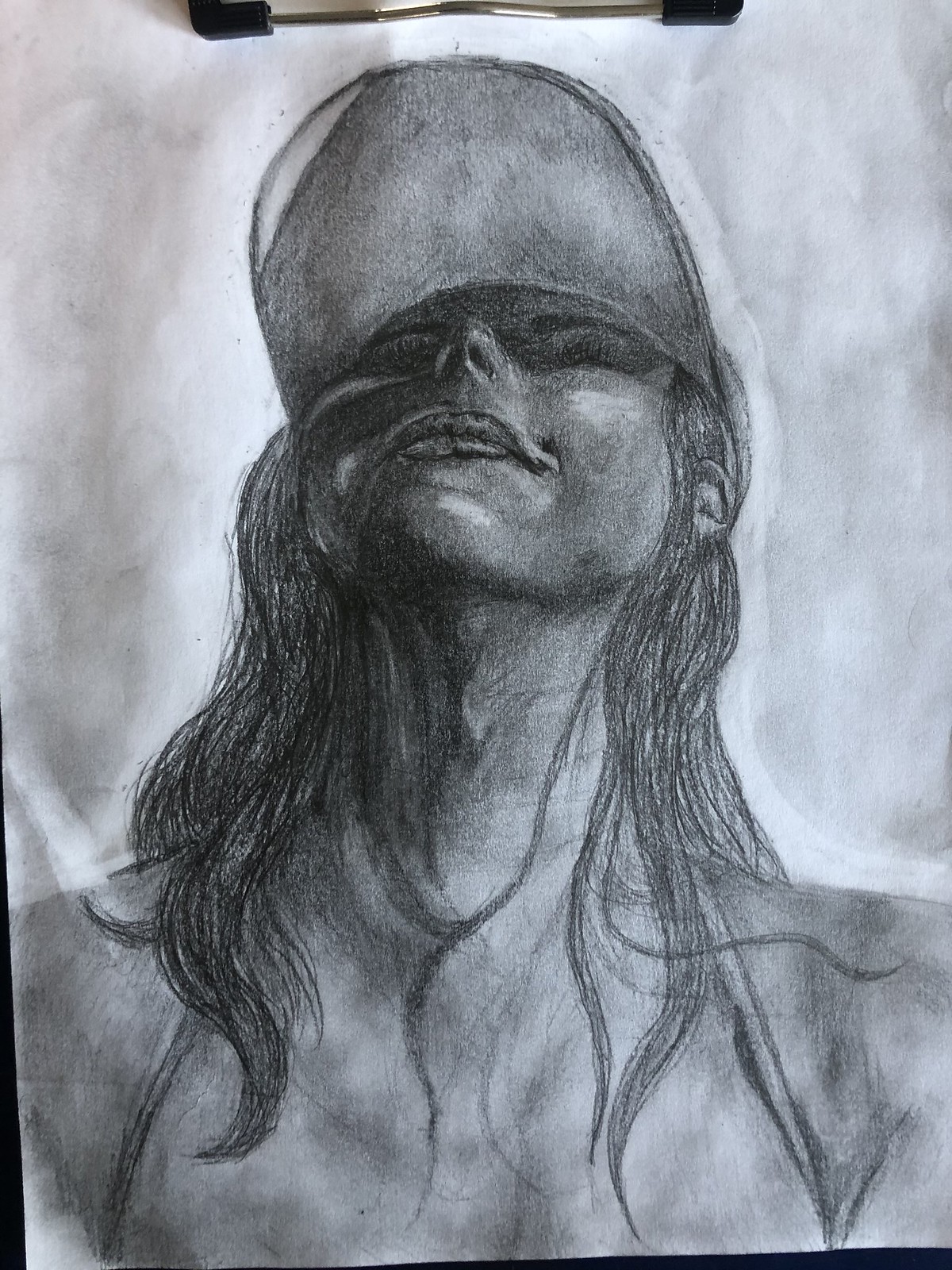The image is a black-and-white photograph of a pencil sketch portraying an upper-torso view of a young woman. The artwork, slightly taller than it is wide, showcases the woman from just above her chest upwards. Her long, dark hair cascades over her shoulders and down her chest, partially concealed under a baseball cap, of which only the underside of the brim is visible. The woman is looking upward at about a 45-degree angle with her eyes closed and lips slightly closed, creating a serene expression. She appears to be in her late teens or early twenties. Her face and body feature detailed shading, with the left side of her neck darker than the right, and the shadows skillfully rendered to emphasize the contours of her features. The background is a light gray, achieved through a subtle smearing effect, typical of a charcoal or pencil medium. The overall scene evokes a sense of calm and introspection, with a meticulously detailed depiction of her long hair and the fine shadows that delineate her facial structure. The image maintains a rough texture around the edges and lacks any text or artist's signature, capturing the raw and unfinished beauty of the sketch.